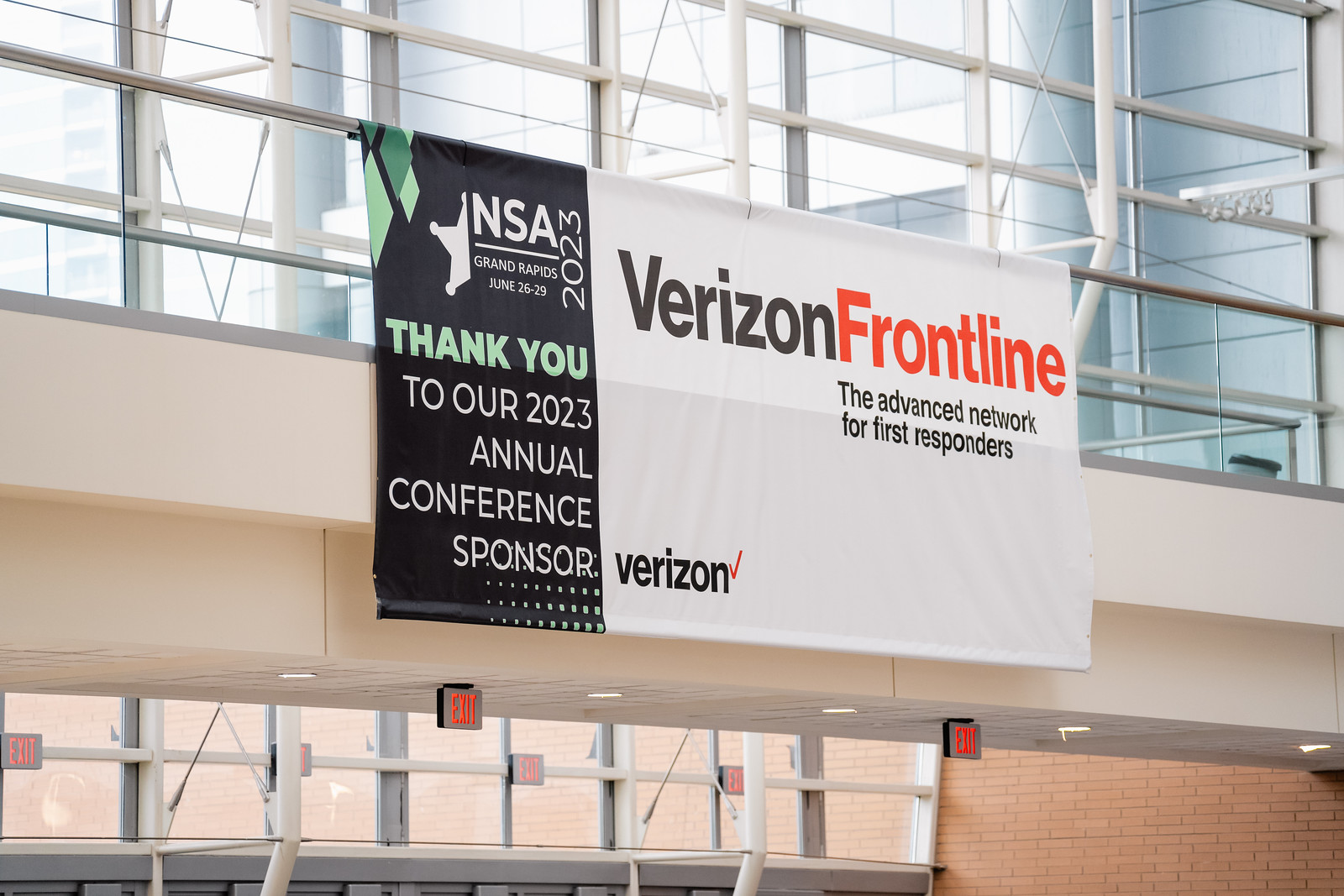The image showcases a banner prominently displayed within a large convention center, likely taken from an upper level. The banner is suspended from a railing above several red-lit exit signs and the tops of doors leading outside. The banner itself is segmented, with the left 25% being black and the rest white. 

On the black section, there's a white logo that says "NSA Grand Rapids 2023." Below it, in green text, it reads "Thank you," followed by "to our 2023 annual conference sponsor" in white. The white portion of the banner features the word "Verizon" in black text, "Frontline" in orange, and beneath it, in smaller black text, "The Advanced Network for First Responders." A black Verizon logo with an orange check mark is placed at the bottom left of the white section. 

The surrounding environment includes silver metal railings, large windows, and either white or metal columns. The lower level displays an orange brick facade on the right, complementing the building's modern architecture and intricate layout.